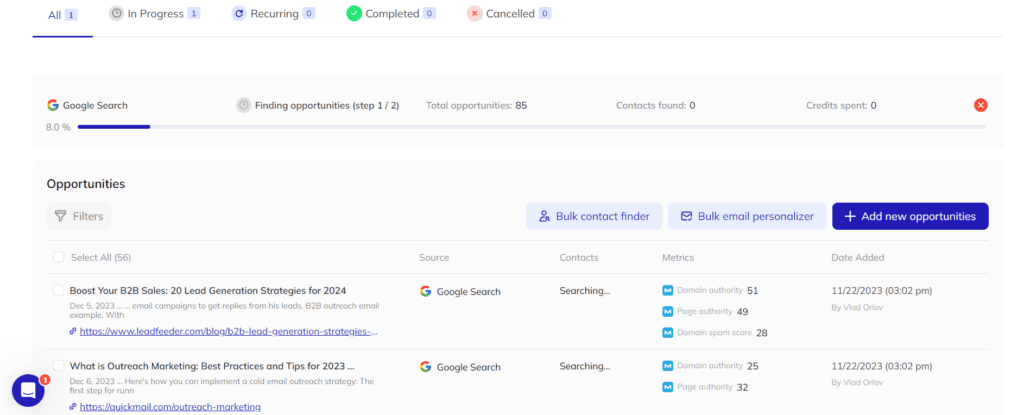### Descriptive Caption:

The depicted web page features a navigation bar at the top with multiple tabs, each accompanied by a numerical indicator within a box. "In Progress" shows a count of 1, while "Recurring," "Completed," and "Canceled" all display a count of 0. Directly below, there's a secondary set of tabs displaying various metrics: "Google Search," "Finding Opportunities," "Step 1 of 2," and "Your Opportunities" with a total count of 85. Additionally, it shows "Contracts Found" at 0, "Credits Spent" also at 0, and a progress bar indicating 8% completion.

Further down, there's a section labeled "Opportunities," featuring a button for "Filters." Within this area, two images and associated links are displayed: 

1. **Boost Your B2B Sales** - featuring "20 Lead Generation Strategies for 2024."
2. **Outreach Marketing Best Practices** - including "Tips for 2023."

Both resources are tagged as sourced from Google Search. The text below provides specific metrics for these links:
- The first link has a domain authority of 51, page authority of 49, and an additional unspecified metric rated 28. This content was added on November 22, 2023, at 3:02 PM.
- The second link shows a domain authority of 25 and a page authority of 32. This content was added simultaneously on November 22, 2023, at 3:02 PM.

The finer details, like the small, light gray text on a white background, capture the intricate metrics of each source.